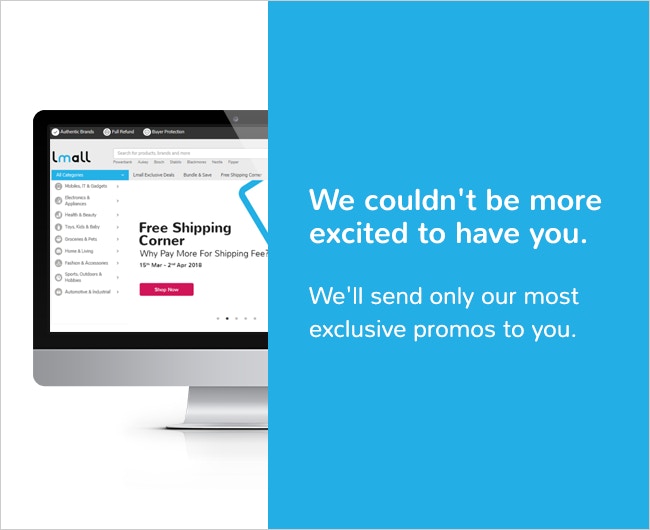This image, captured from a computer screen, is split into two distinct halves: the left side featuring a predominantly white background and the right side highlighted by a light royal blue rectangle. 

**Right Side:** 
- Background: Light royal blue.
- Text Content: 
  - The top sentence, displayed in a larger white font, reads: "We couldn't be more excited to have you."
  - Below, a slightly smaller white font states: "We'll send only our most exclusive promos to you."

**Left Side:**
- Image Display: A silverish computer with a gray front is showcased.
- Screen Content: 
  - Open webpage title: "Free Shipping Corner."
  - Prominent text: "Why pay more for shipping? Why pay more for shipping fee?"
  - Date Range: "15th March to 2nd April 2019."
  - Call to action: A reddish-pink button labeled, "Start Now."
- Sidebar: Contains the text "Elmaw" and a vertical array of clickable icons.

This detailed split-screen image effectively combines promotional messages with a visual representation of a computer screen, inviting user interaction through vibrant and engaging text elements.